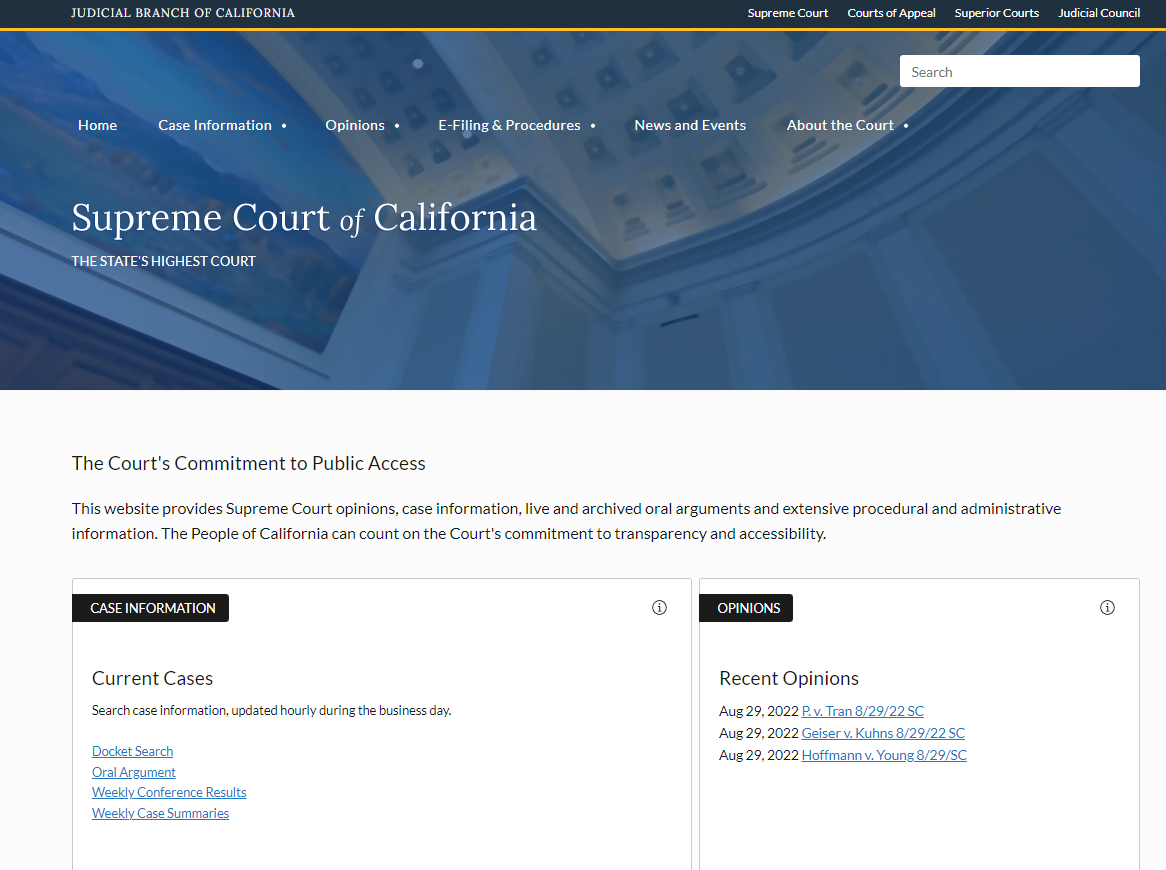This image captures a screenshot of the Supreme Court of California's webpage. Across the top, there is a prominent black horizontal bar featuring white text that reads “Judicial Branch of California: Supreme Court, Court of Appeals, Superior Courts, Judicial Council.” Just below this black section, a thin gold line runs horizontally.

The main background below the gold line is predominantly blue, displaying an image of what appears to be the interior of a courthouse, specifically looking up towards an ornate domed ceiling. Overlaid on this image, white horizontal text provides navigation options including "Home," "Case Information," "Opinions," "E-Filing and Procedures," "News and Events," and "About the Court."

At the center of the page, the title "Supreme Court of California, the state's highest court" is prominently displayed. The blue background subtly transitions from a lighter shade at the top center to a darker tone towards the lower left corner, adding depth and contrast to the overall webpage design.